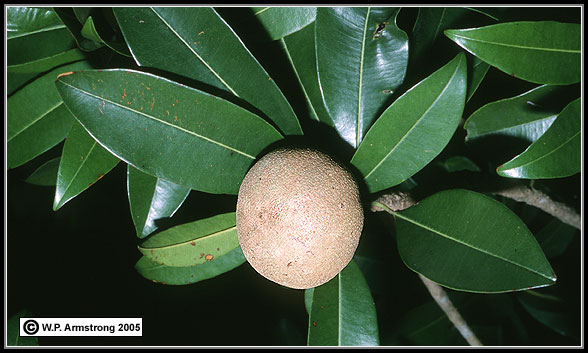The image is a nighttime photograph featuring a central sapodillo fruit surrounded by lush green leaves. The dark background highlights the plant, which is illuminated by a spotlight, making the scene appear almost tropical. The leaves are long, shiny, and waxy, each with a prominent central vein, arranged in a star pattern around the fruit. Brown, thin stalks extend from either side of the frame. The sapodillo fruit, beige to brown in color with a hint of pink, has a rough, textured surface similar to that of a kiwi but without the fur, and is somewhat potato-shaped. The bottom left corner of the photograph includes a copyright notice reading "W. P. Armstrong, 2005" in black text on a white background, adding a touch of authenticity to this representational realism image.